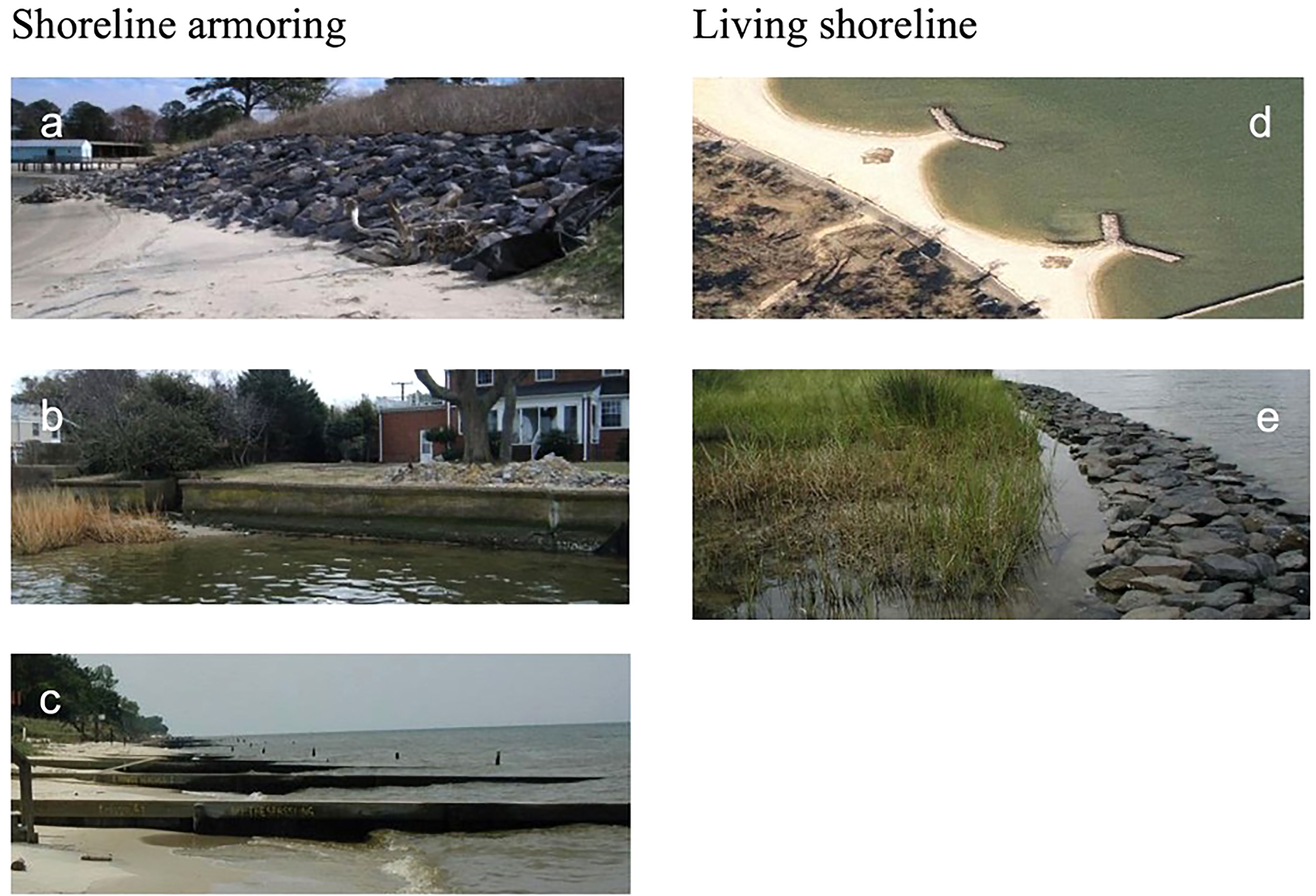The image is a collage of five photographs labeled A through E, arranged in a specific format: three in a column on the left and two on the right, with a blank space in the bottom right. The collage is titled "Living Shoreline" at the top, with the phrase "Shoreline Armoring" written in black letters on a white background just above the left column.

- **Photo A**: Located at the top of the left column, this image depicts a beach area featuring sand, rocks, grass, and trees. The rocks form an incline and are of dark color.
- **Photo B**: Positioned below Photo A, it shows a body of water with greenish-brown hues. There is pom-pom-like grass growing within the water and a levee on the right side. A house and trees are also visible along the coastline.
- **Photo C**: Found at the bottom of the left column, it captures a harbor scene with docks for boats. The water looks dark, and trees are visible along the shoreline.
- **Photo D**: The first photo on the right column is an aerial view displaying water and the coastline.
- **Photo E**: Below Photo D, this image shows more water with numerous rocks around the coastline and patches of grass.

Together, these images illustrate various aspects of shoreline environments and interventions, emphasizing both natural and altered states.